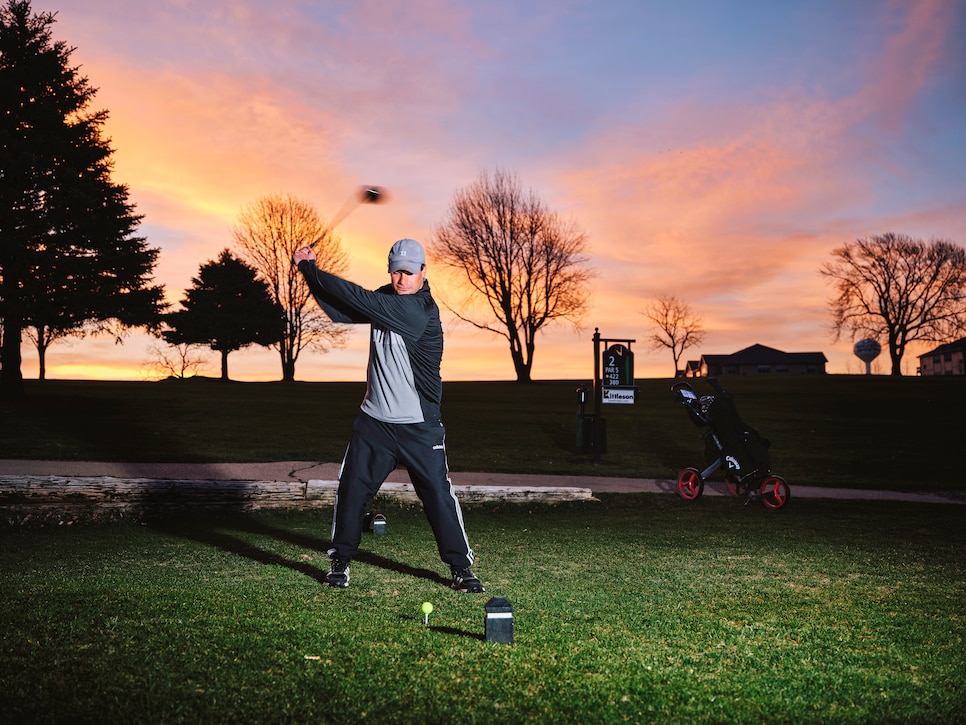In this detailed dusk (or dawn) scene on a golf course, a man dressed in a black and gray tracksuit with a matching gray baseball cap is captured mid-swing with his driver. He’s poised to strike a neon yellow golf ball neatly placed on a white tee, with an additional black box positioned in front of it. The sky overhead features a stunning array of pink and orange clouds, suggesting either a sunrise or sunset.

In the background, a golf club cart with red wheels is visible, along with a sign indicating the second hole. Tall pine trees stand to the left while deciduous trees are on the right, creating a picturesque backdrop. Far off in the distance, several buildings, possibly housing units or a lodge, can be seen. The entire scene is bathed in the soft, fading light of the sky, highlighting the serene and focused atmosphere of the golfer's preparations.